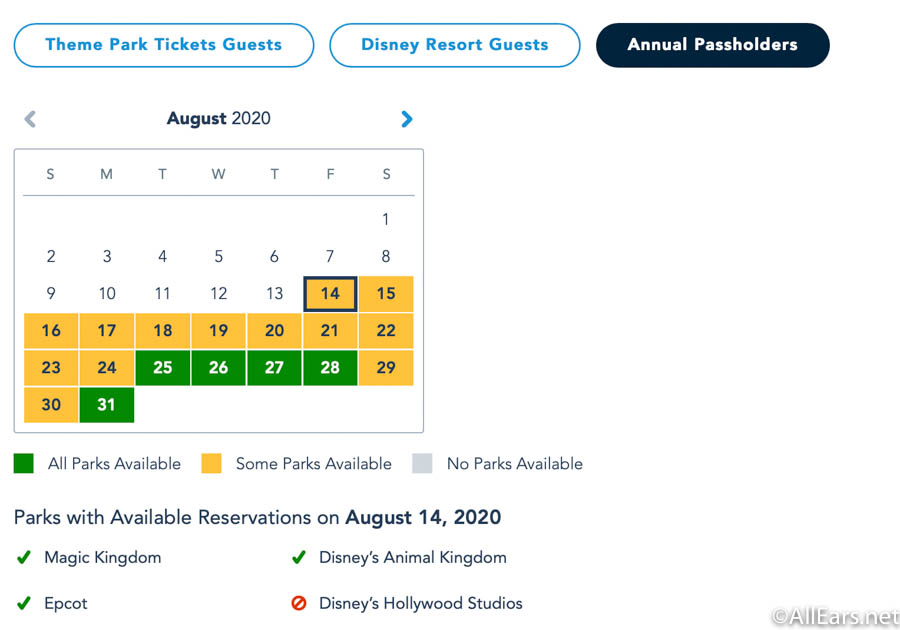The image appears to be a screenshot from the website AllEars.net, featuring a calendar for August 2020 that indicates Disney park availability during the COVID-19 pandemic. The calendar uses a color-coded system to denote park availability: green signifies that all parks are available, yellow indicates that some parks are available, and gray (or white) suggests that no parks are available. Specifically, the dates from the 14th to the 30th are predominantly yellow, with the 25th to the 28th and the 31st marked in green. Notably, Hollywood Studios does not have any available reservations, but Magic Kingdom, Disney's Animal Kingdom, and Epcot do have availability on the green-marked dates. The watermark of the website, displaying AllEars.net, is visible in the bottom right corner, hinting at a possible reference to Mickey Mouse's ears.